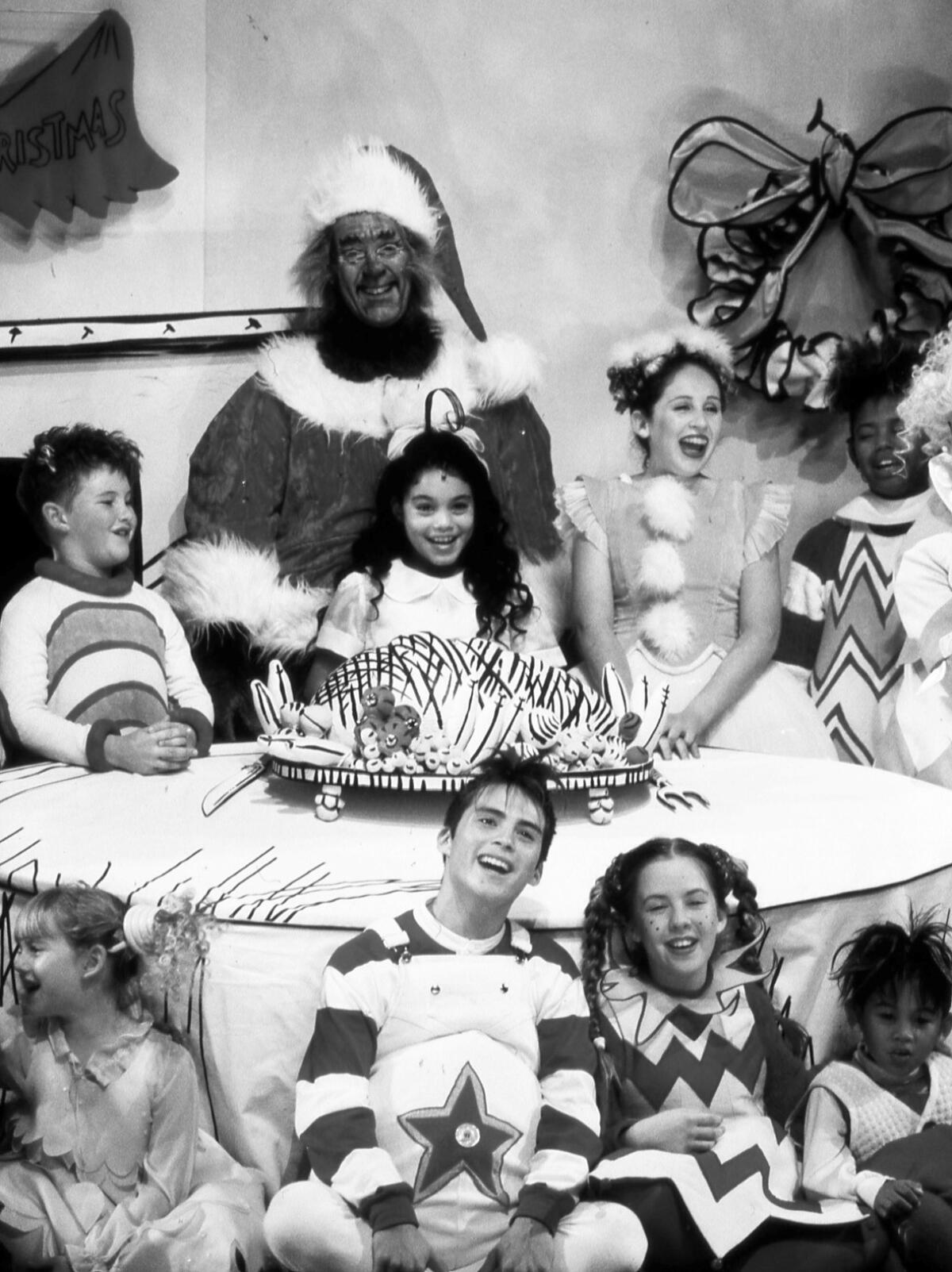This black and white photograph, which appears to be from an old, lower-quality image, captures a lively children’s party with a Christmas theme. At the center and in the back stands an older man dressed as the Grinch, complete with a Santa hat and dark hair sticking out underneath, but without the traditional white beard. Next to him, there's an adult female with red lipstick and a full smile, adorned in an outfit with white poofy buttons and matching puffs on her head. In front of this pair, eight children are captured in varying costumes, many displaying bold patterns. 

To the right of the Grinch, a little boy in a striped shirt and animal ears is noticeable, standing next to a girl in a simple white dress. Another girl beside her wears a costume dress with a fluffy wig. To her right is a boy in an outfit with zigzag stripes. In the front row, seated alongside a table laden with dishes, another group of children is visible. On the left, a little girl sits; next to her, a taller boy with white suspenders, adorned with a star, laughs at the camera. Beside him, a girl in a zigzag-patterned outfit with pigtails and freckles on her face smiles, as does a baby next to her. The festive atmosphere is enhanced by a partially visible “Christmas” banner and a wreath in the background. The children’s joy radiates through their smiles, capturing the essence of a joyous holiday celebration.